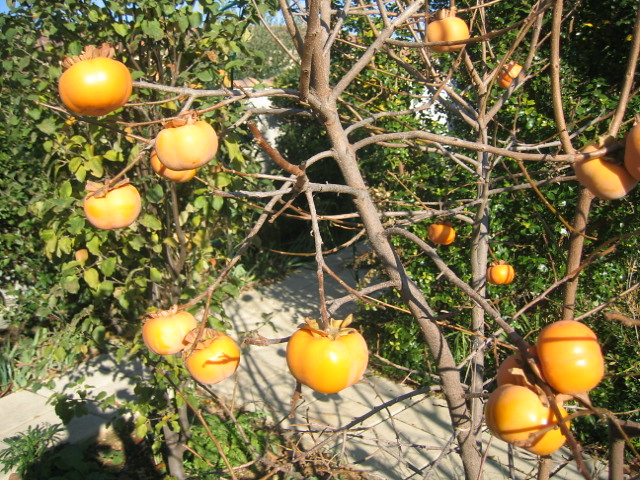This close-up color photograph showcases a persimmon tree with bare, woody branches adorned with numerous ripe fruits resembling tomatoes. These persimmons are deep golden-yellow to yellowish-orange, indicating their peak ripeness. The tree stands prominently in the foreground along a concrete path that forks and leads into wooded areas. Surrounding the persimmon tree are other lush, green trees, with glimpses of a body of water and patches of blue sky peeking through the foliage. The vivid scene is captured on a sunny day, with the leafless persimmon tree and its distinctive fruits providing a striking contrast to the verdant and leafy background.